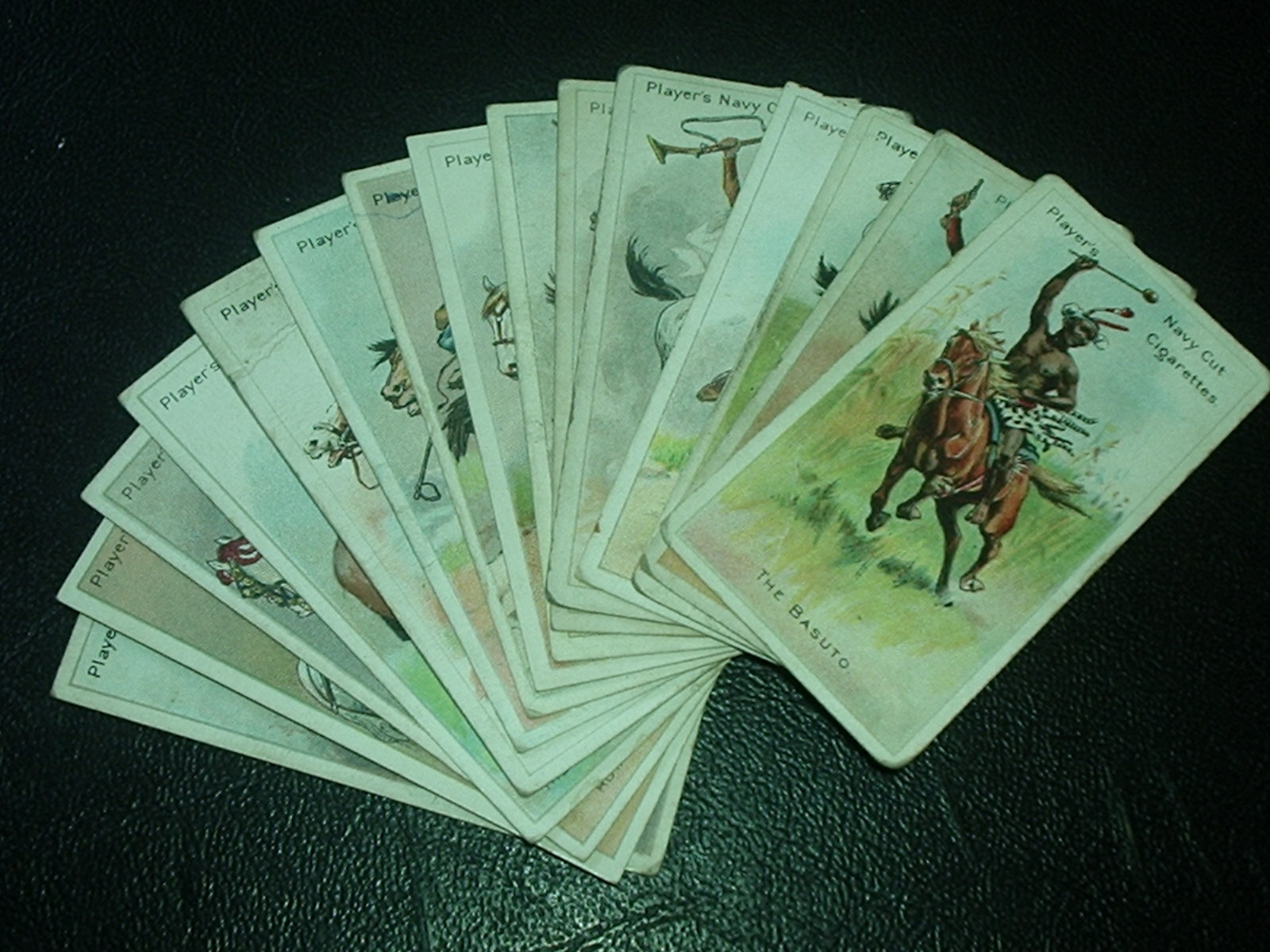A set of 15 playing cards is displayed on a shiny black pebbled leather background. Arranged in a fan-spread pattern as if held in hand, the cards appear to be promotional items. The topmost card prominently features "Players Navy Cut Cigarettes" at the top and "The Basuto" at the bottom. The artwork on the back of the card depicts a dynamic scene: a brown pony with a light brown mane and tail, galloping through a lush green field. Riding the pony is a person with black skin, dressed in a black and white loincloth patterned with spots. The rider, holding the reins in their left hand, has their right arm raised high, gripping a stick with a large bulbous end. Their head is adorned with white flowers and two long, thin decorations, possibly feathers or plant stems, extending from the back and arching over their head. The rider is seemingly enjoying the high-speed ride, exuding an air of exhilaration.